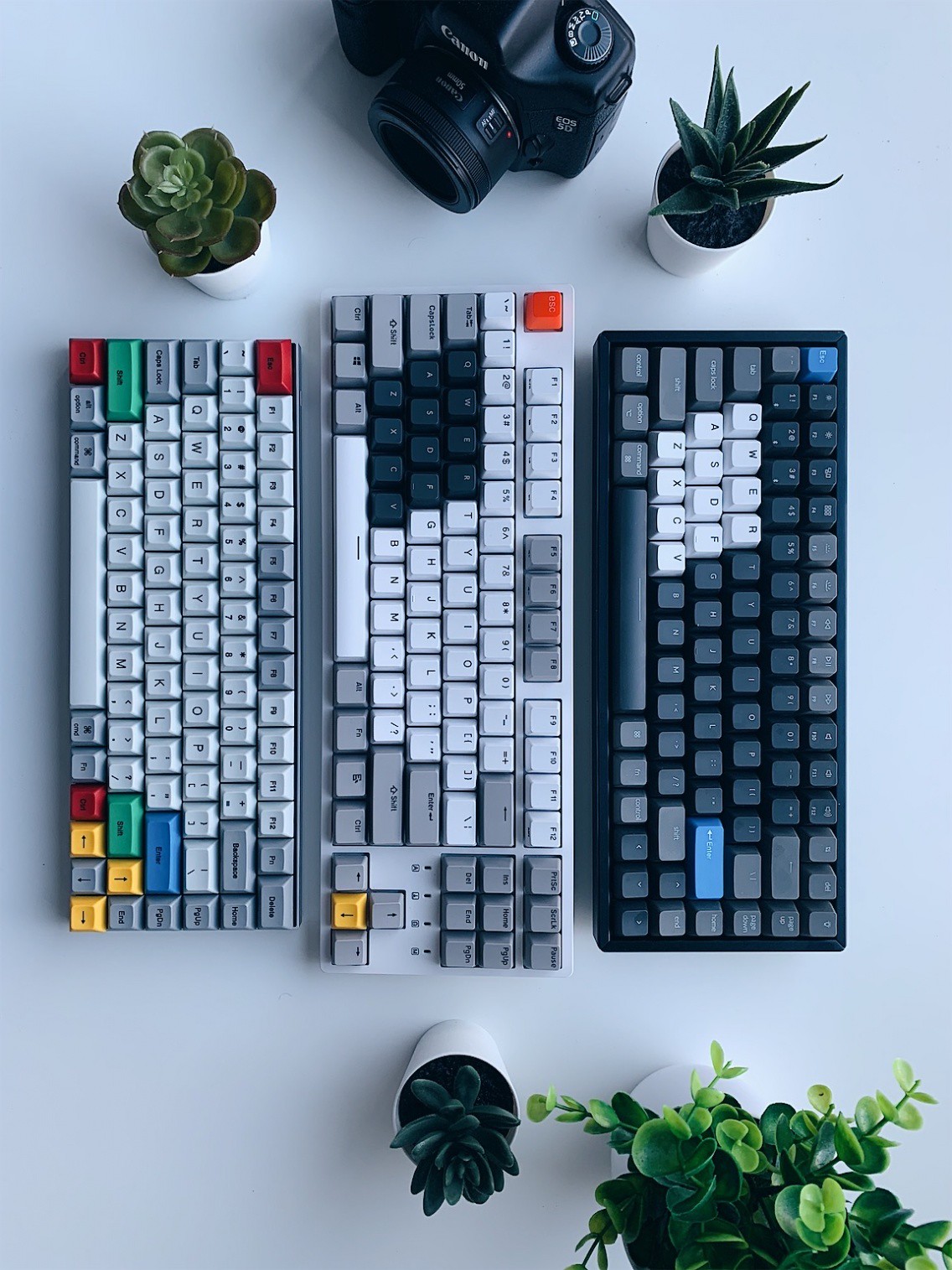The image showcases a light blue desktop adorned with various objects in an organized manner. Starting from the bottom, there is a white tabletop featuring two potted plants; the smaller pot houses a green succulent, and the larger pot contains a cactus. Centrally aligned in the image are three mechanical keyboards arranged vertically. The leftmost keyboard is compact, predominantly white, featuring a collection of colorful keys. The middle keyboard stands out as a full-sized gaming keyboard with black keys, notably having the WASD cluster in darker contrast. The rightmost keyboard is again compact, predominantly black, with the QWERASDF and ZXCV keys distinctly highlighted in white. Moving towards the top of the image, a DSLR Canon camera is positioned centrally between the keyboards, flanked by another set of potted plants; a cactus on the upper left and an aloe plant on the upper right complete the scene, evoking a balanced mixture of technology and nature.